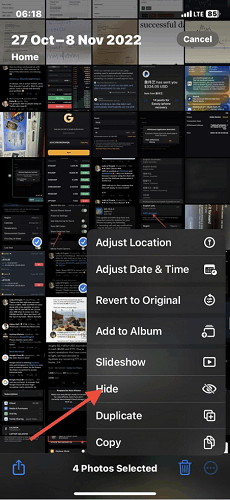This image is a cropped screenshot from a mobile phone's camera roll. The primary background consists of thumbnails for various screenshots and photos. At the very top left corner, the text "27 October to 8 November 2022" is prominently displayed in bold white letters, signifying the date range for the images shown. Below that, in smaller white letters, the word "home" is visible, indicating the current screen tab. To the upper right-hand corner, there's a grey button labeled "Cancel" in white text.

At the bottom right of the screenshot, a pop-up box is visible, containing a vertical list of options. The option "Hide" is highlighted, and a red arrow, edited onto the photo, points directly to it. This indicates the user's intent to hide certain photos. Across the lower part of the screenshot, it shows that four photos have been selected for hiding. 

To the far left side, there is a share button, while on the far right, there are a trash can icon and a circular menu option. The menu option is currently selected, which explains the appearance of the pop-up box at the bottom right. 

Finally, at the very top left of the screenshot, time information is visible, displaying "6:18." To the top right, status icons including a signal strength indicator, an LTE symbol, and a battery icon complete the status bar details, offering a comprehensive view of the device's current status.